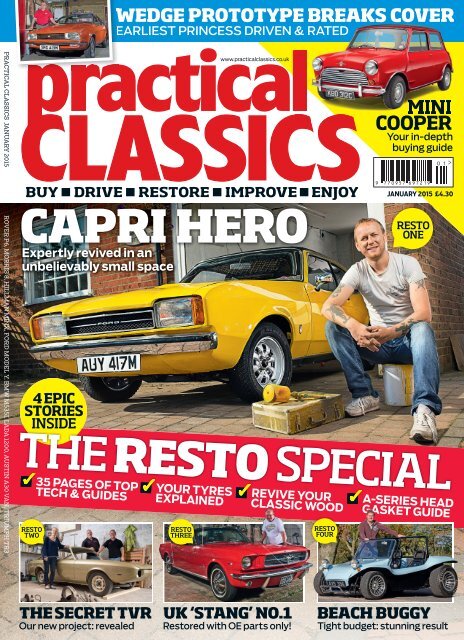This is the front cover of a brightly colored motor enthusiast magazine called Practical Classics. The magazine title is prominently displayed in red at the top with the subtitle "Buy, Drive, Restore, Improve, Enjoy" in black text beneath it. A blue banner at the very top reads "Wedge Prototype Breaks Cover, Earliest Princess Driven and Rated" in white text.

The main feature is an article titled "Capri Hero, Expertly Revived in an Unbelievably Small Space," accompanied by a large image of a yellow muscle car. A man dressed in a white t-shirt, jeans, and white sneakers is sitting on a paint bucket with his hands clasped together beside the car. 

A red banner in the middle of the cover declares it a "Resto Special," highlighting 35 pages of top tech and guides. Further details include segments such as "Your Types Explained," "Revive Your Classic Wood," and "Series Head Gasket Guide."

At the bottom of the cover are three images of different vehicles labeled as "The Secret TVR," "UK Stang Number One," and "Beach Buggy." Additionally, there are six cars pictured on the cover: two red cars, a yellow car, an orange car, a gold car, and a light blue beach buggy. The design uses loud, bold fonts and is packed with various details about classic and modern cars.